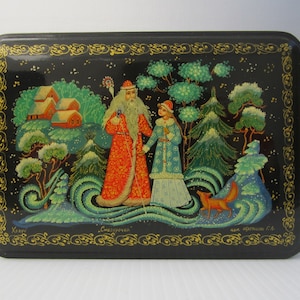The image depicts a detailed, hand-stamped rectangular box set against a white background. The box itself is black with a gold, lacy ornate border surrounding an intricate illustration. The scene on the box shows an older man dressed in a flowing red robe and hat, suggestive of Saint Nick or a wizard, holding a long staff. He stands beside a young girl clad in a blue robe and sweater. They are amidst a winter landscape with snow on the ground, which flows like waves. In the background, there are snow-covered trees and houses under a night sky. To the right, a small animal, possibly a fox or a dog, can be seen. The overall color tones are predominantly black, gold, red, blue, orange, and green. The illustration style is ornate and somewhat abstract, capturing a magical, festive scene within its design.